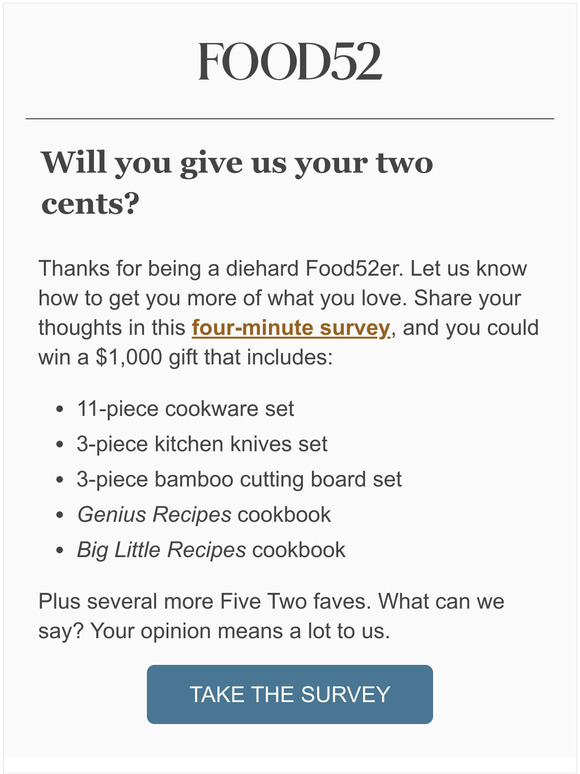This is a detailed and polished caption for the provided description:

---

The image is a screenshot of a pop-up ad from Food52, encouraging users to take a survey. The background is light gray, and at the top, the brand name "FOOD52" is displayed in dark gray, all-caps, in an elegant font. Directly beneath this, a thin light gray line separates the header from the main content. A prominent dark gray heading reads, "Will you give us your two cents?" 

Below this, in standard dark gray 12-point font, the text thanks users for their loyalty: "Thanks for being a die-hard Food52-er. Let us know how to get more of what you love. Share your thoughts in this four-minute survey." The phrase "four-minute survey" is highlighted in gold and underlined.

Further enticing participation, the ad mentions a $1,000 gift prize. The prize details include: 
- 11-piece cookware set
- 3-piece kitchen knife set
- 3-piece bamboo cutting board set
- Genius Recipes cookbook
- Big Little Recipes cookbook
- Several more 5-2 favorites

The ad concludes with a phrase emphasizing the value of user feedback: "What can we say? Your opinion matters to us." Below this is a prominent call-to-action button in dark teal-gray with white text that reads, "Take the survey."

---

This version provides a structured and detailed description of the pop-up ad with clear attention to text hierarchy and visual elements.